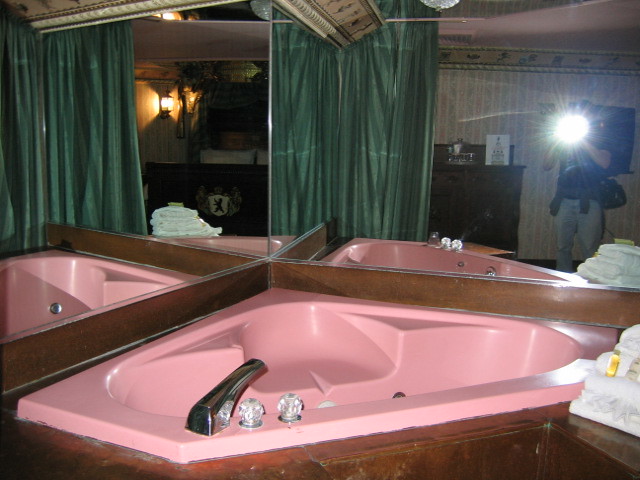This photograph depicts a unique interior space, likely a bathroom, centered around a vintage pink pentagon-shaped whirlpool tub, reminiscent of the popular 50s style. The tub, framed with dark wood, features clear acrylic knobs and a chrome faucet. Positioned in a corner, the tub is surrounded by wall-to-wall mirrored surfaces, which multiply its image and the details of the room, creating an intricate play of reflections. 

In the mirrors, a green curtain is visibly drawn, along with an ornate cream ceiling, and striped wallpaper with a decorative border. The reflections also reveal various elements of the space; a brown dresser, a wall sconce, and a neat stack of folded white towels on a brown built-in counter. The mirrors reflect the pink tub three times, intricately layering the deep tub’s seat and dual crystal knobs within the mirrored surfaces.

Additionally, a person photographing the room is partially visible in the reflections. Dressed in light jeans and a short-sleeve shirt with a gray sweatshirt around their waist, only their arms and the bright flash from their camera are discernable. This creates an intriguing visual where reality melds with its mirror images, capturing the room's elegant retro aesthetic and its layered, almost kaleidoscopic effect.